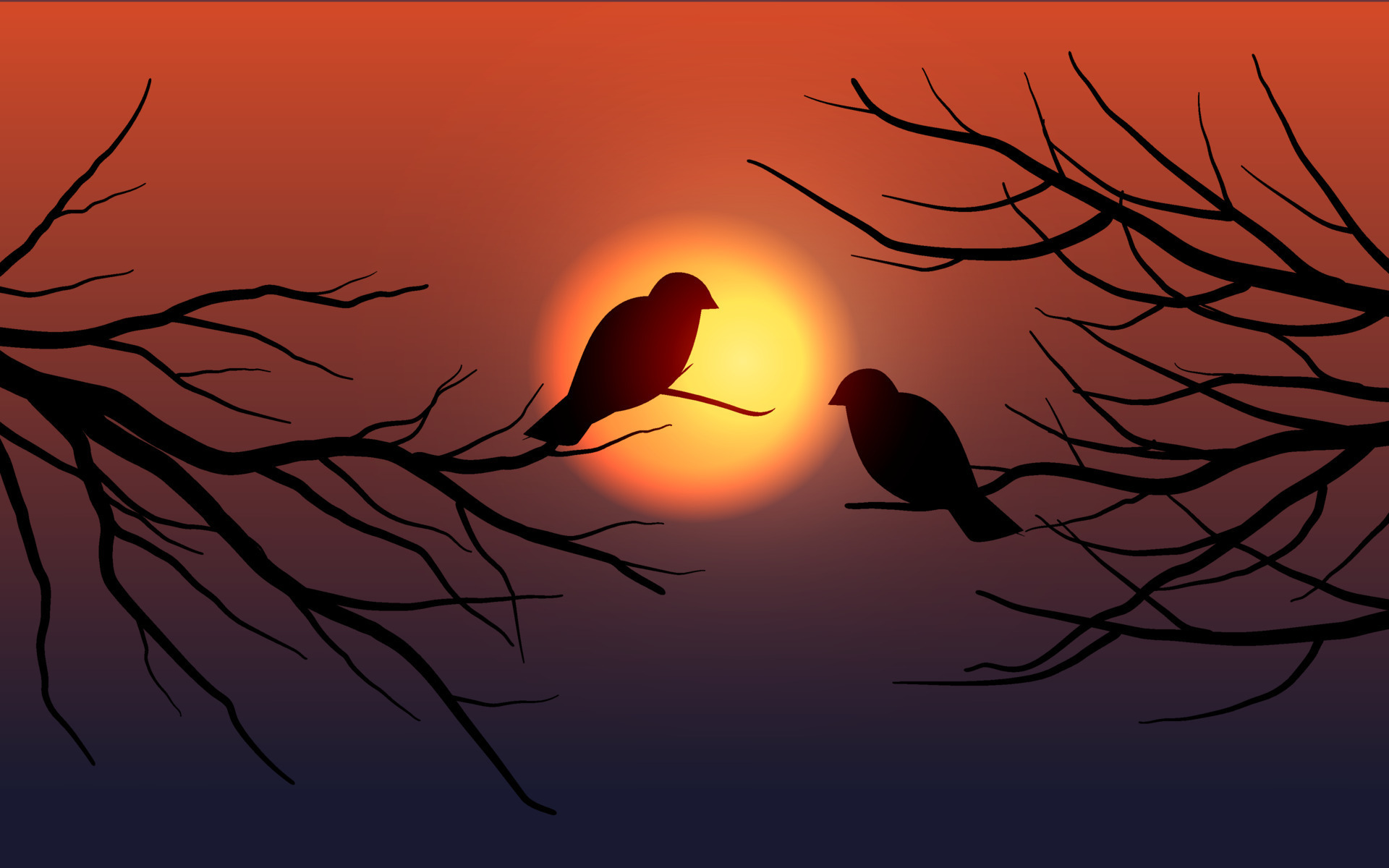This digital painting, likely a color illustration, captures a tranquil sunset scene. At its center is a hazy, dim golden sun, featuring a yellow core and an outer rim tinged with orange, casting a warm glow across the sky. The sky itself transitions through rich gradients of red, orange, brown, and dark purple. Silhouetted against this vivid backdrop are two dried-up tree branches extending from either side of the image. Perched on these branches, slightly askew from each other, are the shadowy figures of two small birds, possibly sparrows or ravens. The bird on the left branch sits higher, directly in front of the setting sun's center, while the lower bird on the right branch gazes back at its companion. This evocative scene, rendered in landscape orientation, uses contrasting elements of black silhouettes and colorful gradients to emphasize the serene yet haunting beauty of the moment.